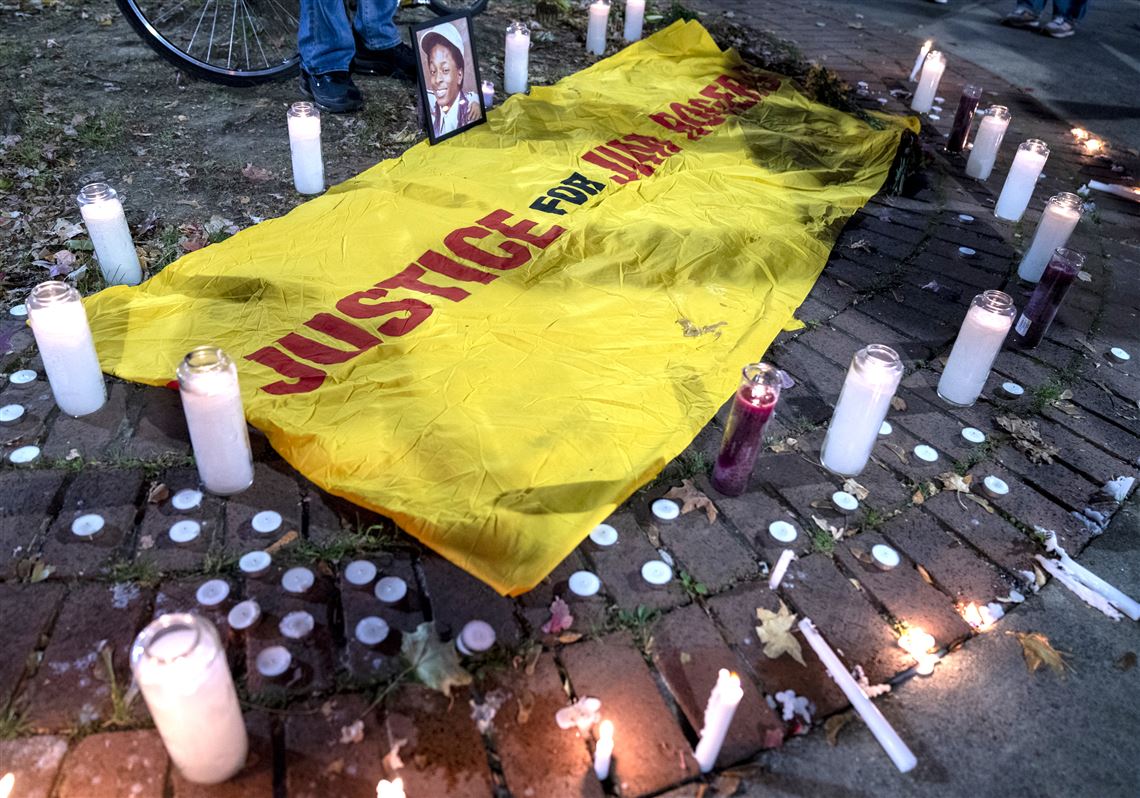The photograph depicts an outdoor memorial, likely used at a vigil for Jim Rogers, a victim of violence. The centerpiece of the image is a yellow flag laid on the brick ground, prominently displaying the words "Justice for Jim Rogers" with "Justice" and "Jim Rogers" in red text and "for" in black text. At the top of the flag, there is a picture of a young boy, presumably Jim Rogers. This image is encircled by an arrangement of tall white pillar candles, with additional red and black tall candles interspersed among them. Tea candles are scattered throughout the scene, some lit and some extinguished, adding to the solemn atmosphere. In the background, the lower half of an individual wearing jeans and sneakers is visible, along with a bicycle wheel on the left side. The setting appears to be a park, with other people present at the periphery of the photo, making the scene one of communal mourning and tribute.